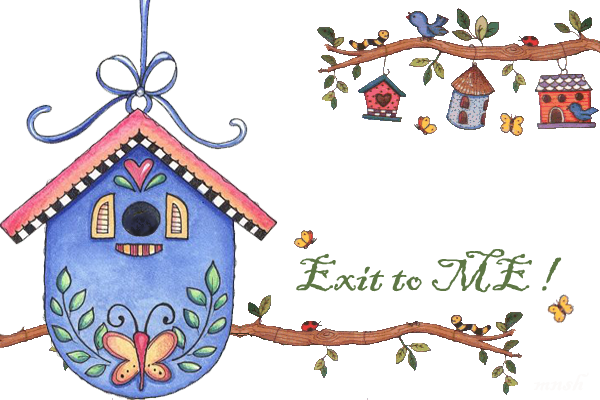In this image, a vibrant blue birdhouse stands to the left, adorned with an intricate design. A red and yellow butterfly with green leaves on either side decorates the bottom of the birdhouse. Above the birdhouse's entrance is a red heart, and its roof features black and white checkered lower sections with pink-orange shingles. Nearby, yellow shutters add to the picturesque scene.

To the right of this birdhouse, a branch with various insects and leaves extends into the frame. The branch hosts caterpillars, butterflies, and ladybugs amidst its green foliage. In the upper right corner, a detailed depiction of three birdhouses hangs from another branch: a square birdhouse with a black interior heart-shaped window, contrasting blue roof and red sidewalls decorated with black polka dots; a cylindrical birdhouse with a brown roof and blue sides featuring dotted patterns and four brown doors; and a traditional birdhouse with a blue and white roof, a red body, and a blue bottom, with a blue bird peeping in.

The leftmost birdhouse, suspended by a blue ribbon, has a pink roof with black and white stripes below, blue walls, and a pink heart above the entrance. Yellow and white shutters, green leaves on black stems, and a red and yellow butterfly complete its facade. Accompanying these charming birdhouses are more butterflies, caterpillars, ladybugs, and green leaves. The entire scene, set against a white background, bursts with color: blue, pink, red, yellow, and green dominate the palette. Additionally, the text "Exit to Me!" in green is prominently featured above the branch, adding an animated and whimsical touch to the lively and colorful tableau.